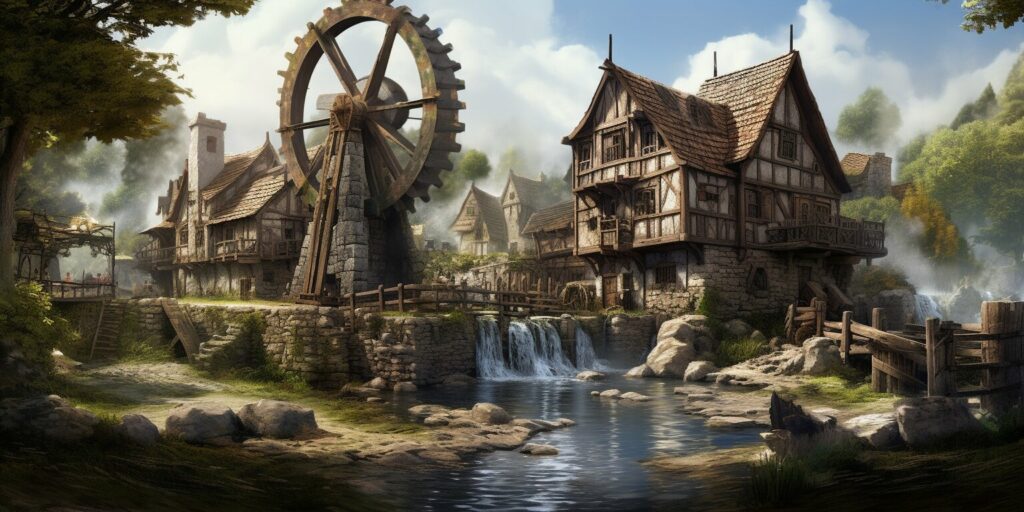The image depicts a highly realistic painting set in what appears to be a medieval landscape. In the foreground, a small waterfall cascades down a rocky, green terrain, blending seamlessly with patches of gray stone and lush grass. Towering trees frame the scene on both the upper left and right corners, their foliage creating a natural border. The sky above is a serene expanse of blue, dotted with fluffy white clouds, adding a tranquil atmosphere to the setting.

To the right of the waterfall stands an old-fashioned watermill, characterized by its large, greenish-brown wheel and sturdy brick base tinged with gray. The mill is juxtaposed with several traditional medieval houses, predominantly brown with white accents, lending an air of historical authenticity to the scene. The intricate details and carefully rendered elements evoke the simplicity and rustic charm of medieval times, capturing a moment of serene beauty in a bygone era.